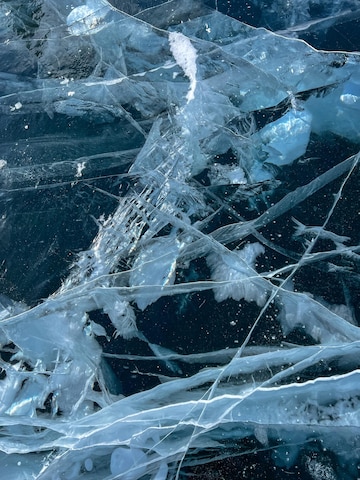A high-resolution color photograph captured in natural light depicts a close-up view of a sheet of ice, characterized by its intricate patterns of cracks and fissures. The ice exhibits a spectrum of dark and light blues, creating a striking contrast against the translucent areas through which one can glimpse the water beneath, suggesting a frozen lake or pond. Jagged cracks of varying sizes stretch horizontally and vertically without any discernible pattern, with some being noticeably larger in the foreground. Embedded within the ice are what appear to be organic materials, possibly leaves, feathers, and twigs, all frozen in place and giving the impression of a brittle, glass-like surface. The absence of marine life, coupled with the visible depth of the cracks and woven organic materials, creates a mesmerizing snapshot of nature in a delicate state of freeze, as if capturing the moment just as the water solidifies.